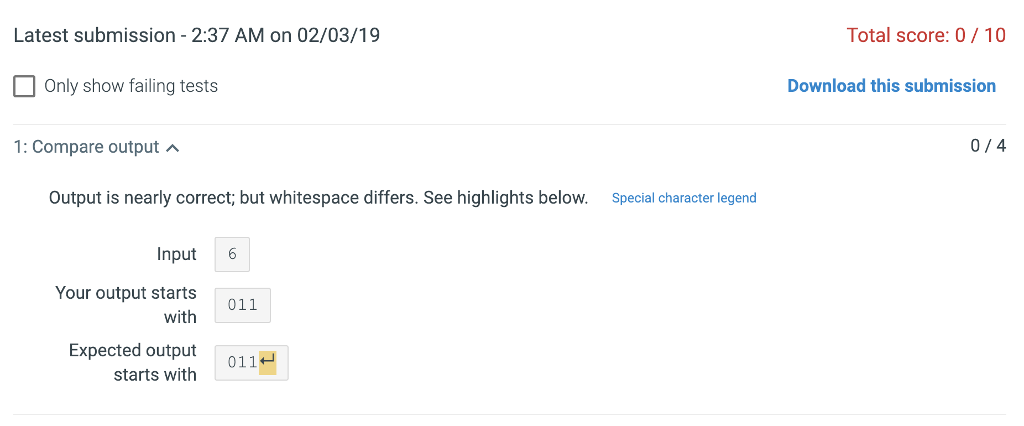This screenshot captures a widescreen, landscape-oriented view of a testing platform interface. At the top of the screen, a banner reads "Latest submission: 2.37 a.m. on 02.03.19," alongside a total score of "0 out of 10." A checkbox labeled "Only show failing tests" is visibly unchecked. To the right, there is a button labeled "Download this submission." 

Further down, informative text states, “One compare output. Output is nearly correct but whitespace differs. See highlights below.” Adjacent to this text, there's a button for a "Special Character Legend."

In the main section, a box labeled "Input" shows the value "6" as the provided input. Another section displays "Your Output," which begins with "0 1 1," and "Expected Output," which also starts with "0 1 1," followed by an arrow symbol suggesting a comparison between the two outputs.

This image seems to be analyzing a failed test submission, with detailed markers to help the user understand the discrepancy, primarily focusing on whitespace differences in the output. The presence of functionality for downloading the submission and highlighting specific issues indicates that this is a comprehensive tool for developers or testers aiming to debug and refine their code submissions. Without additional context, it is challenging to determine the exact nature of the test, but the interface is clearly designed to facilitate detailed examination and correction of coding errors.